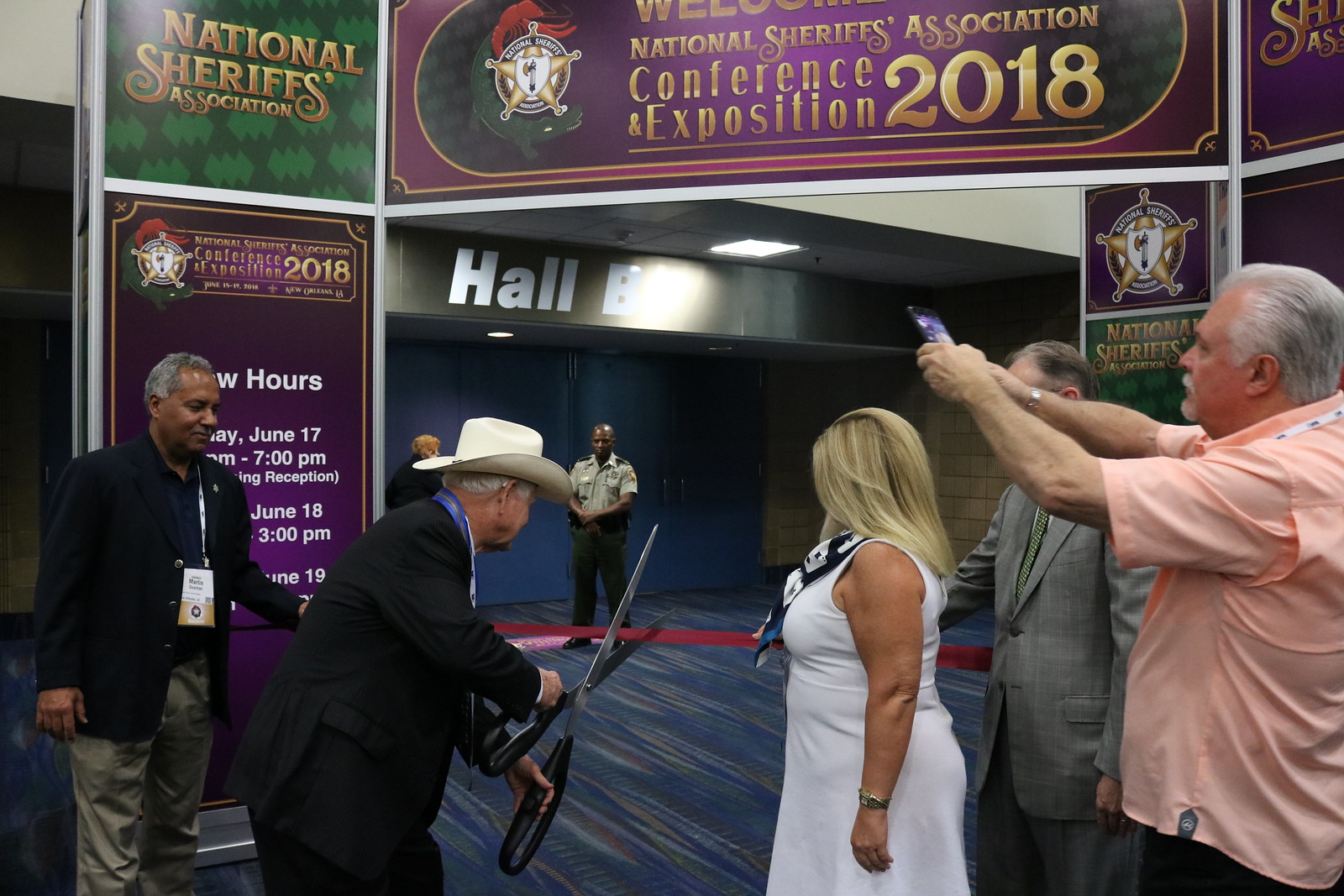In this vibrant color photo, a ribbon-cutting ceremony for the National Sheriffs Association Conference and Exposition 2018 is taking place. The red ribbon is stretched between an archway adorned with posters that read "National Sheriffs Association Conference Exposition 2018" and "Welcome National Sheriffs Association Conference Exposition 2018." Central to the scene is a man in a suit and a bright white cowboy hat, poised to cut the ribbon with an oversized pair of scissors. To his left stands another man in a suit jacket and khakis, wearing a lanyard. On his right, a blonde woman in a white dress is positioned next to an older gentleman in a gray suit and another older man in a peach short-sleeved shirt, who is holding his phone high to capture the moment. The backdrop includes four blue double doors and a security guard beside someone else near the entrance. The venue's carpet features a wavy pattern of blue, green, brown, and lighter green hues.